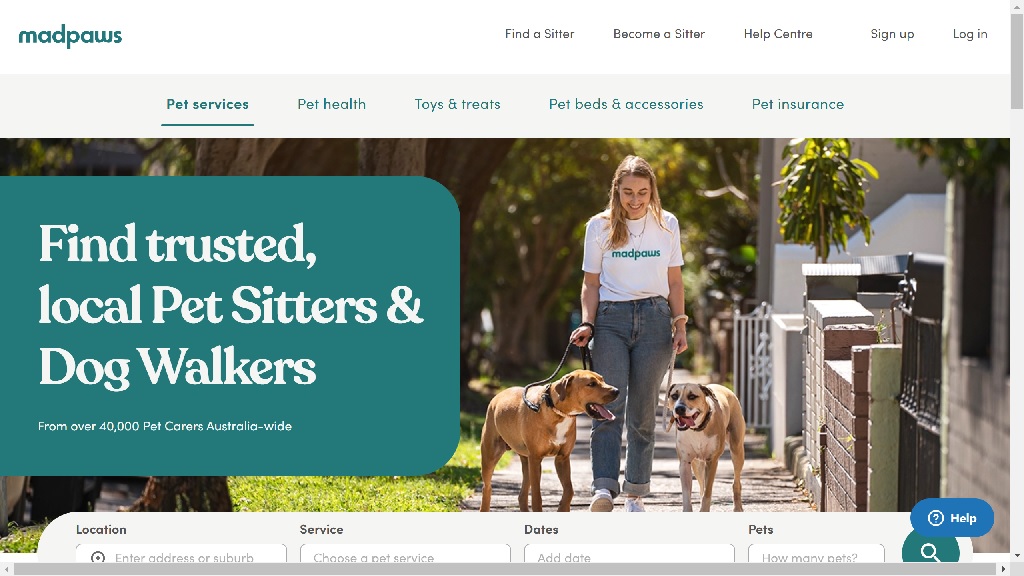In this image, we see a well-structured web page dedicated to pet services. The web page features a clean white background. On the upper left corner, there is a green logo with the text "Mad Paws." Moving from left to right across the top, you'll find grey text links for "Find a Sitter," "Become a Sitter," "Help Center," "Sign Up," and "Log In." There is also a grey box with an upward pointing arrow next to these links. A darker grey bar runs along the top, with a lighter grey bar extending down to the arrow at the bottom.

In the center of the page, a light grey background features a blue title with an underlined blue text that reads "Pet Services." Below this, a horizontal navigation menu goes from left to right, listing "Pet Health," "Toys and Treats," "Pets," "Beds and Accessories," and "Pet Insurance."

Further down, on the left side, a green background with white font states, "Find Trusted Local Pet Sitters and Dog Walkers from over 40,000 pet carers Australia-wide." Just below, against a grey background with black font, are form fields labeled "Location," "Service," "Dates," and "Pets." Each field provides specific instructions: "Enter Address or Suburb" for Location, "Choose a Pet Service" for Service, "Add a Date" for Dates, and "How Many Pets?" for Pets.

On the right side, there's a distinctive blue circle with a white question mark labeled "Help," followed by a green circle with a white magnifying glass icon that says "Search."

The image prominently features a person walking two dogs, illustrating an example of the service offered. The person, who has long brown hair and is wearing a white Mad Paws t-shirt, grey-blue jeans, and white running shoes, is walking along a tree-lined sidewalk. The two dogs, one dark brown and the other light brown, are on leashes. The surroundings include green grass and gated walls on either side of the pathway.